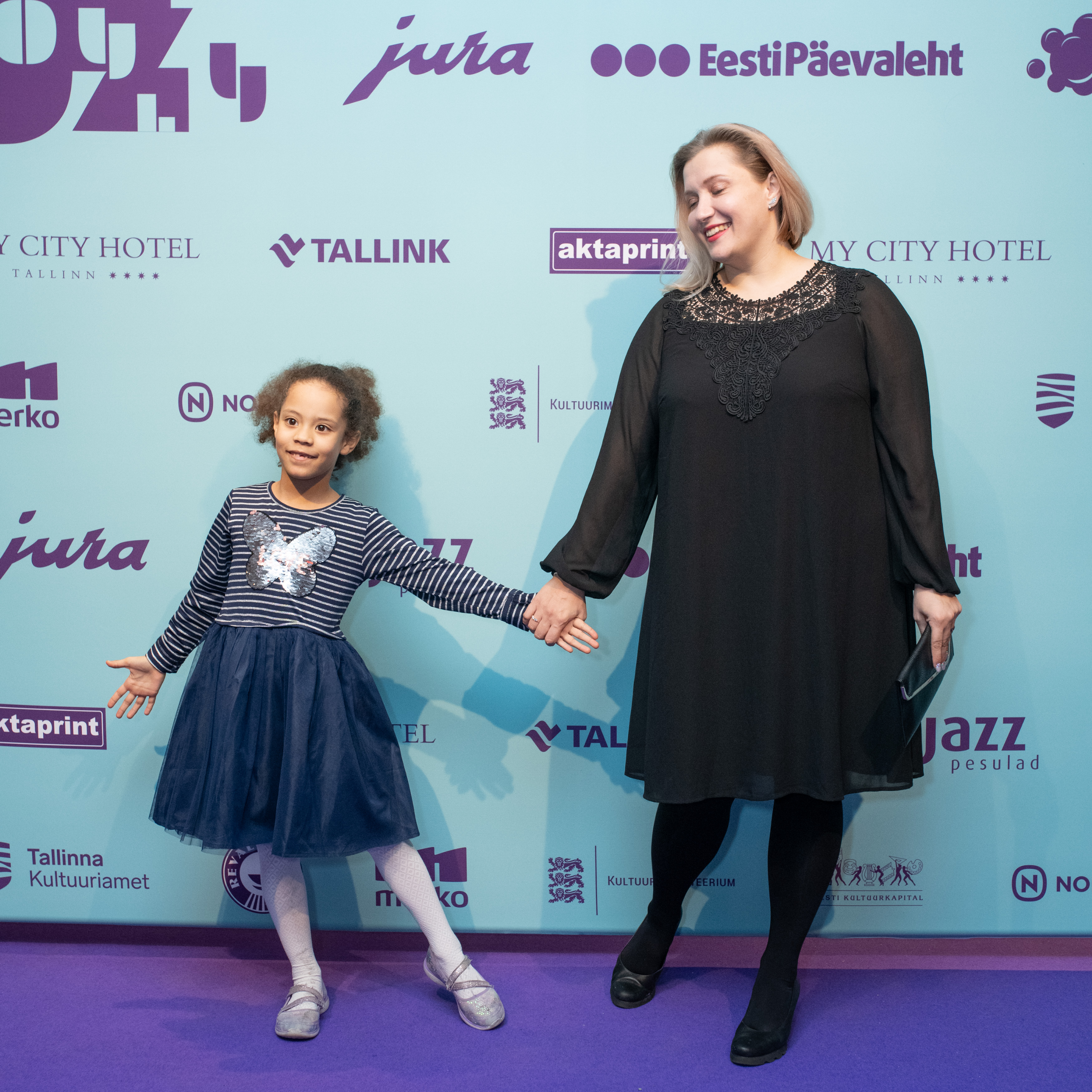The photograph captures a touching moment between a smiling blonde woman and a young African-American girl, who are holding hands while standing on a purple-carpeted runway, commonly used for photo ops at events. The background wall is light turquoise, adorned with various sponsor logos, including "Jiro," "Tall Inc," "ActiPrint," and "My City Hotel." 

The woman, whose blonde hair falls to her shoulders, is depicted in a black dress featuring a lace top, accompanied by black stockings and shoes. She accessorizes with a small purse and radiates a warm smile, enhanced by her red lipstick, though her eyes are closed as she gazes down at the girl.

The young girl, with caramel-toned skin and curly hair tied back, is exuberantly dressed in a navy blue and white striped long-sleeved shirt with a shiny silver butterfly design on the front. She pairs this with a frilly, pleated navy-blue skirt, white stockings, and ballet slippers. The girl's dark eyes and beaming smile add to the charm of the image, making this moment both memorable and heartwarming.